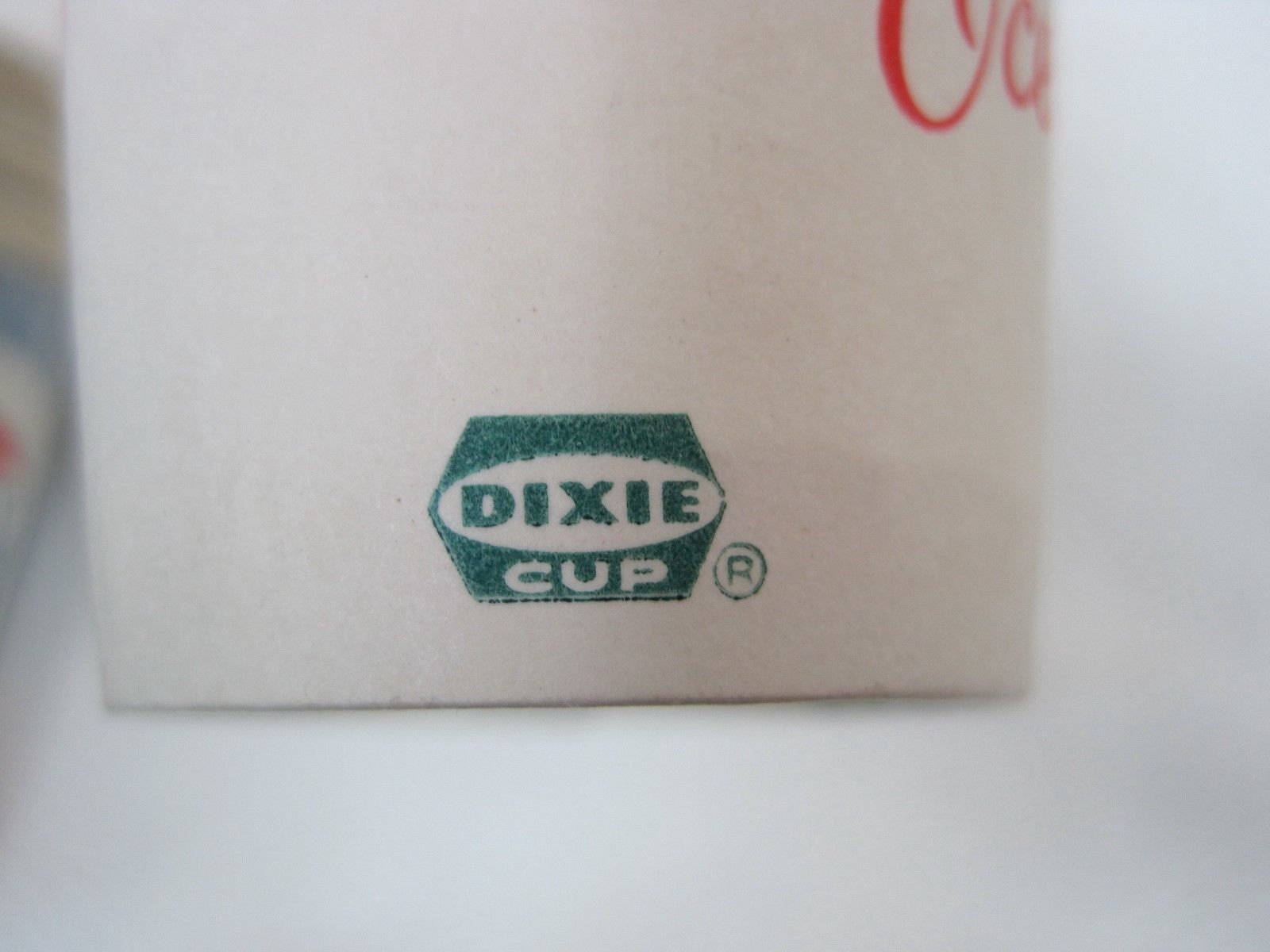In this close-up color photograph, the primary focus is on the bottom of a white Dixie cup, although the entire cup is not visible. The distinctive Dixie cup logo is prominently featured, comprising a white oval within a dark green elongated shape. Inside the oval, the word "Dixie" is written in dark green text, while below it, "C-U-P" is displayed in white text on the green background. Adjacent to the text is a small "R" in a circle, indicating the registered trademark. The cup is positioned slightly off-center to the top left, with some unreadable orange-red text visible on its right side. The background is a silvery grey, implying an ambiguous setting, possibly a counter or even a trash bin. The image is largely monochromatic with brief hints of other colors, including blue, tan, and red, visible in the blurred background.